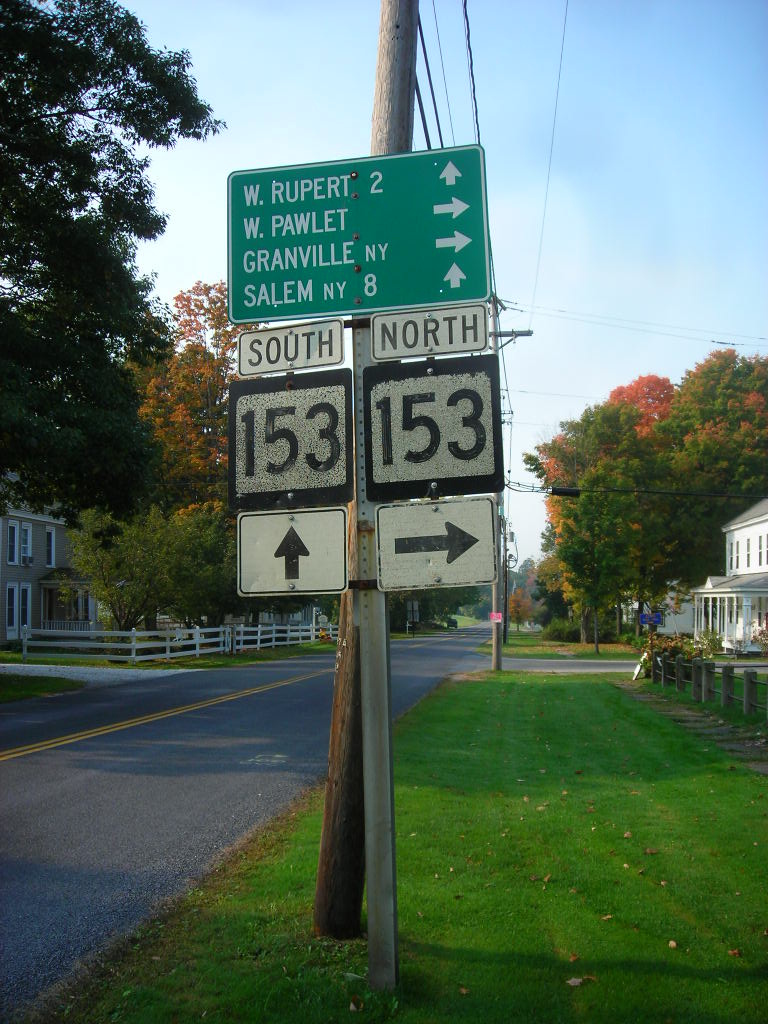A photograph captures a quaint, sunlit street scene. The vibrant blue sky is sprinkled with a few soft clouds, setting a cheerful backdrop. The street is a two-lane road marked by dual yellow lines running down its center. On either side of the road, meticulously maintained green grass frames the scene, leading up to charming, older two-story buildings. The building to the right is painted white, while the one on the left appears to be constructed of stone, though its details are somewhat obscured.

Prominently featured in the image is a street sign atop a metal pole. The topmost sign, with a green background and white lettering, reads "W. Rupert 2" with an upward-pointing arrow. Below it, another green sign directs "W. Paulette" to the right. The third sign points right towards "Granville, New York," followed by a fourth sign that reads "Salem, New York 8" with an arrow pointing straight ahead.

At the bottom, a sign indicates "South 153" with an arrow pointing straight ahead, while to its right, another sign directs "North 153" with an arrow pointing right. A brown telephone pole behind the sign is adorned with various wires, adding to the rustic charm of the scene.